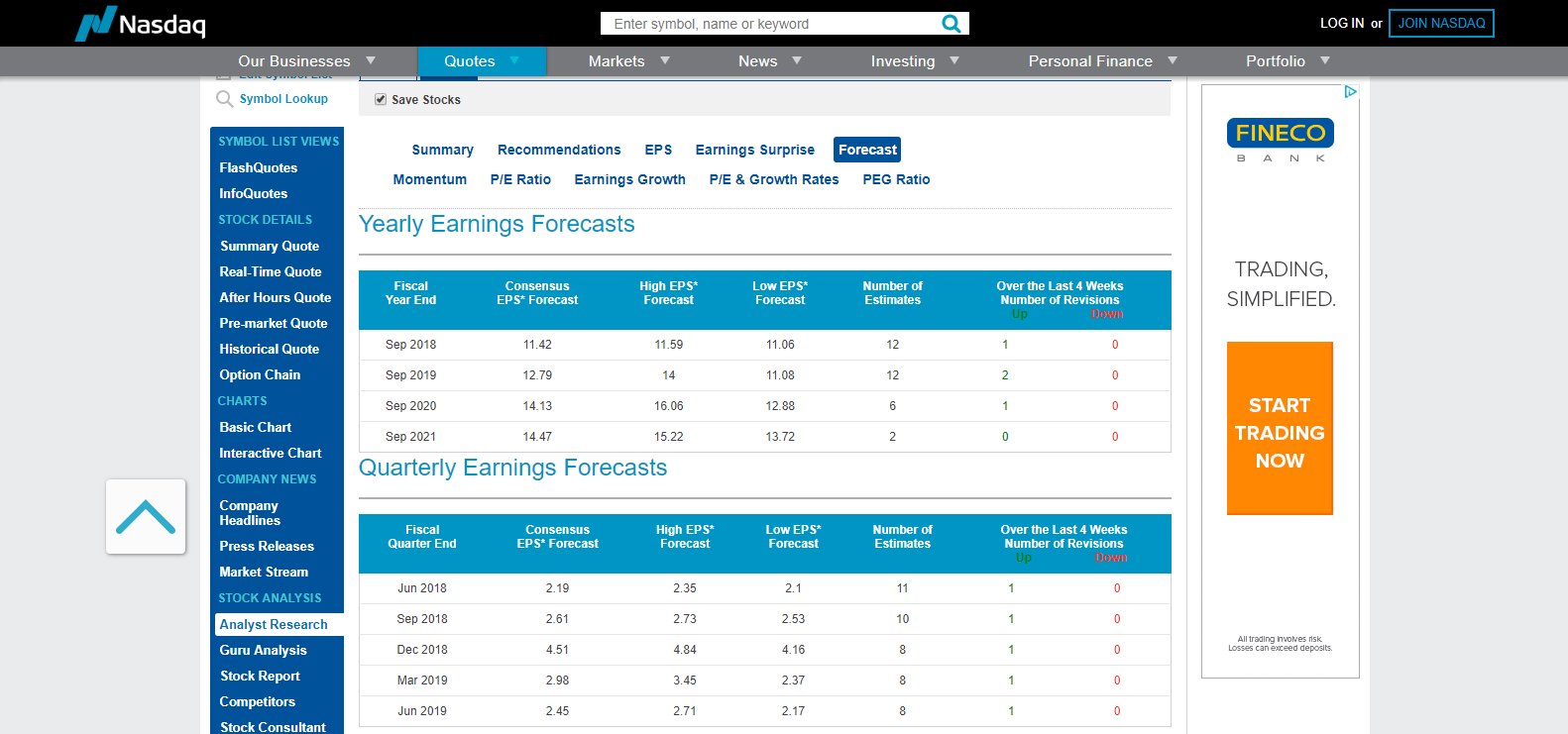The image is a screenshot from the NASDAQ website, resembling the layout of a spreadsheet with organized rows and columns. Along the left side, it displays a variety of options, including symbols and a "Symbol Lookup" feature. Key headers visible in the middle section include "Symbol," "Last," "List Views," and "Flash Quotes," followed by "Info Quotes," "Stock Details," "Summary Quote," "Real-Time Quote," "After Hours Quote," and "Pre Market Quote."

Continuing down, the menu expands with choices like "Historical Quote," "Option Chain," and various charting tools such as "Basic Chart" and "Interactive Chart." Further sections feature "Company News," "Company Headlines," and "Press Releases," along with "Market Stream," "Stock Analysis," and "Analyst Research."

The focal point of the screenshot is the "Analyst Research" section. Here, the user has clicked on "Forecast," specifically viewing the "Yearly Earnings Forecast" section. This area details the "Fiscal Year," "Consensus EPS Forecast," "High EPS Forecast," "Low EPS Forecast," and the "Number of Estimates." Additionally, it outlines "Number of Revisions" over the past four weeks, supplemented by two charts illustrating these figures.